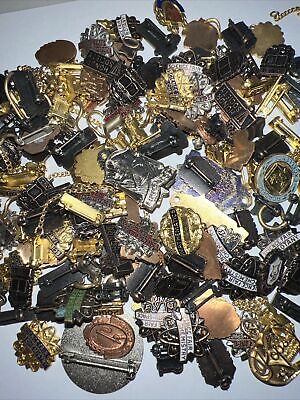The image is a full-color, vertically rectangular photograph taken indoors under artificial light, capturing roughly 30 to 50 metallic trinkets scattered across a light blue surface, which appears white in some descriptions likely due to lighting. These trinkets include brooches, pins, and lapel-like items, many of which have inscriptions and engravings that are too small to read. The designs vary, featuring images such as trains and boats, as well as shapes resembling shields and official seals. Predominantly, these items are made of brass, showcasing colors like gold, copper, silver, and black, with some pieces potentially being plastic. The trinkets are arranged in random positions, with some prominently displaying their intricate fronts while others show only their backs, all gleaming under the lighting.